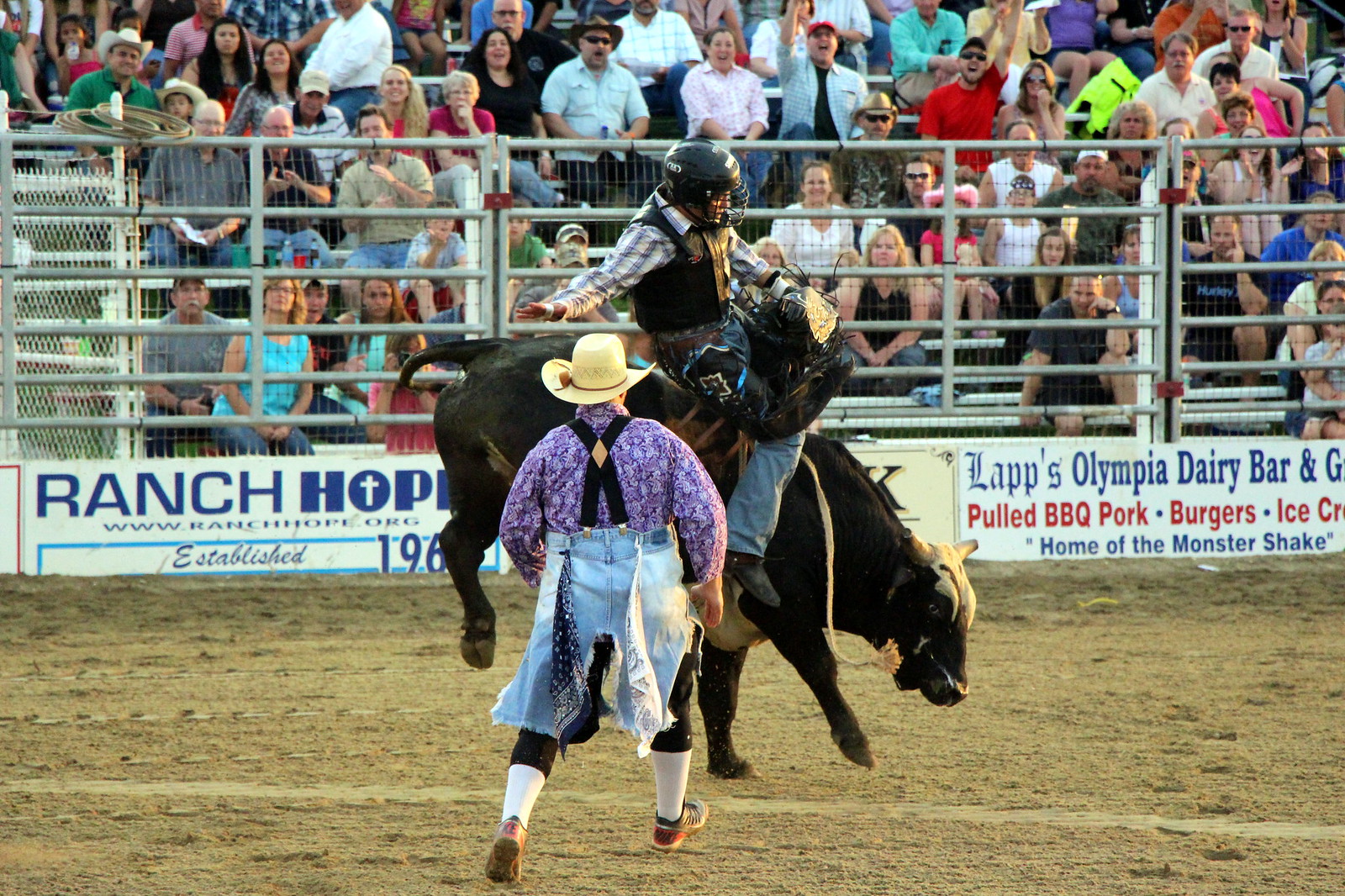This dynamic rodeo scene captures the excitement of the event, set against a packed backdrop of enthusiastic spectators. In the center of the image, a cowboy is riding a violently bucking bull, struggling to maintain his balance with one arm outstretched. He’s dressed in a black vest, a striped long-sleeve shirt, blue jeans, and a helmet resembling a football helmet. Below, a rodeo clown in a colorful purple paisley shirt, baggy torn jeans, white socks, and a straw cowboy hat is running towards the bull, attempting to distract it. Surrounding the dirt arena, a metal fence separates the spirited audience from the action, with several advertising signs visible, including Ranch Hope and Laps Olympia Dairy Bar, which offers Pulled Barbecue Pork, Burgers, Ice Cream, and the Monster Shake. The crowd, behind the railing, is a mix of cheerful, excited, and intensely watching spectators.